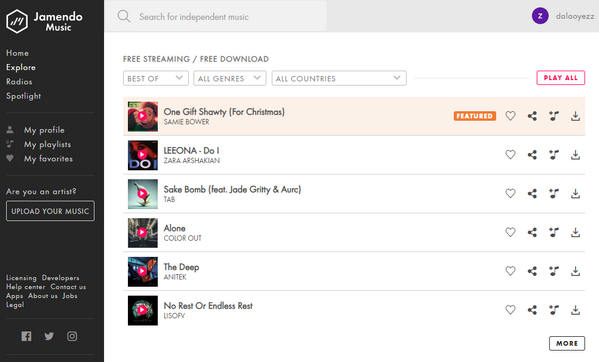The image features a user interface titled "John Mendo Music" in the top left corner. The navigation menu includes options such as Home, Explorer, Radio, Spotlight, Persons, My Profile, My Playlist, My Favorites, Are You An Artist, Upload Your Music, Licensing, Developers, Help Center, Contact Us, Apps, Bias, Jobs, Legal. Social media icons for Facebook, Twitter, and Instagram are also present.

The search bar allows users to look for Independent Music. Highlighted artists and features include Deloyer Yez, Saint Bauer, and OneGearShotty with a Christmas-themed release. Other highlighted names are Paula Del Hart, Cher Bun, Leona Dwyer, Sarah Arkshan, and Jade Grady. The interface mentions various functionalities such as free streaming and free downloads.

Some of the featured collections and playlists include "Best of," "All Drums," "All Country," and a prominently displayed "Orange Rectangle featuring Paula Del Hart, Cher, and Succubong." The description also references a restaurant named D&O Restaurant, with a casual phrase, "Let's Rest," possibly indicating a pause or break feature in the music streaming service.